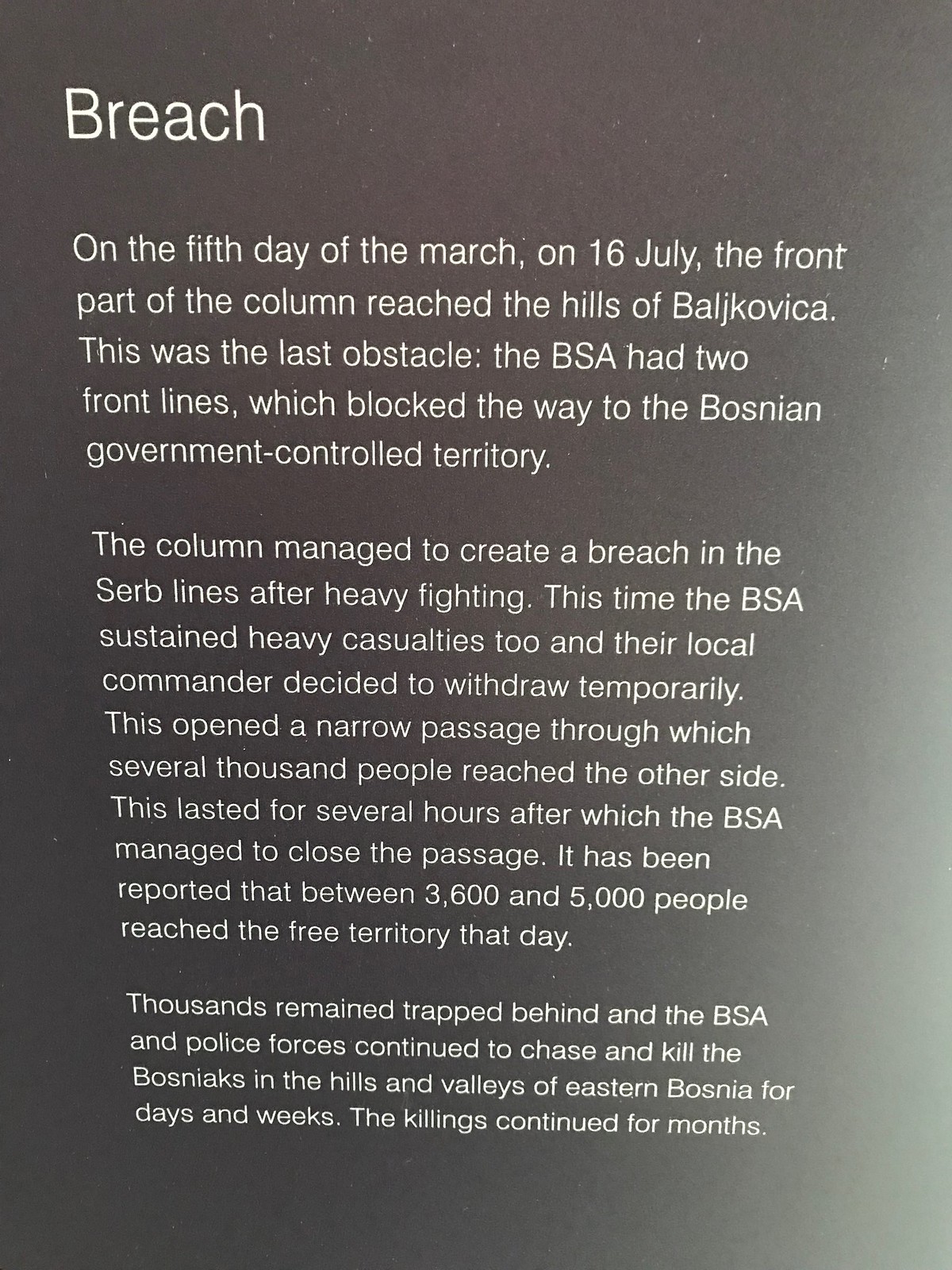The caption for the image could read:

"The sign, set against a gradient of grey to black, prominently displays the capitalized word 'Breach' at the top in a larger font. Below the title, the white text narrates a critical event: 'On the fifth day of the march, July 16th, the front part of the column reached the hills of Belakovia, encountering the last obstacle. The Bosnian Serb Army (BSA) had two front lines blocking the route to Bosnian government-controlled territory. After heavy fighting, the column created a breach in the Serb lines. Despite sustaining heavy casualties, the BSA's local commander ordered a temporary withdrawal, opening a narrow passage. This allowed several thousand people to cross to the other side over several hours before the BSA sealed the passage. Reports indicate that between 3,600 and 5,000 people reached free territory that day. However, thousands remained trapped. The BSA and police forces continued to pursue and kill Bosniaks in the hills and valleys of eastern Bosnia for days, weeks, and even months.'”